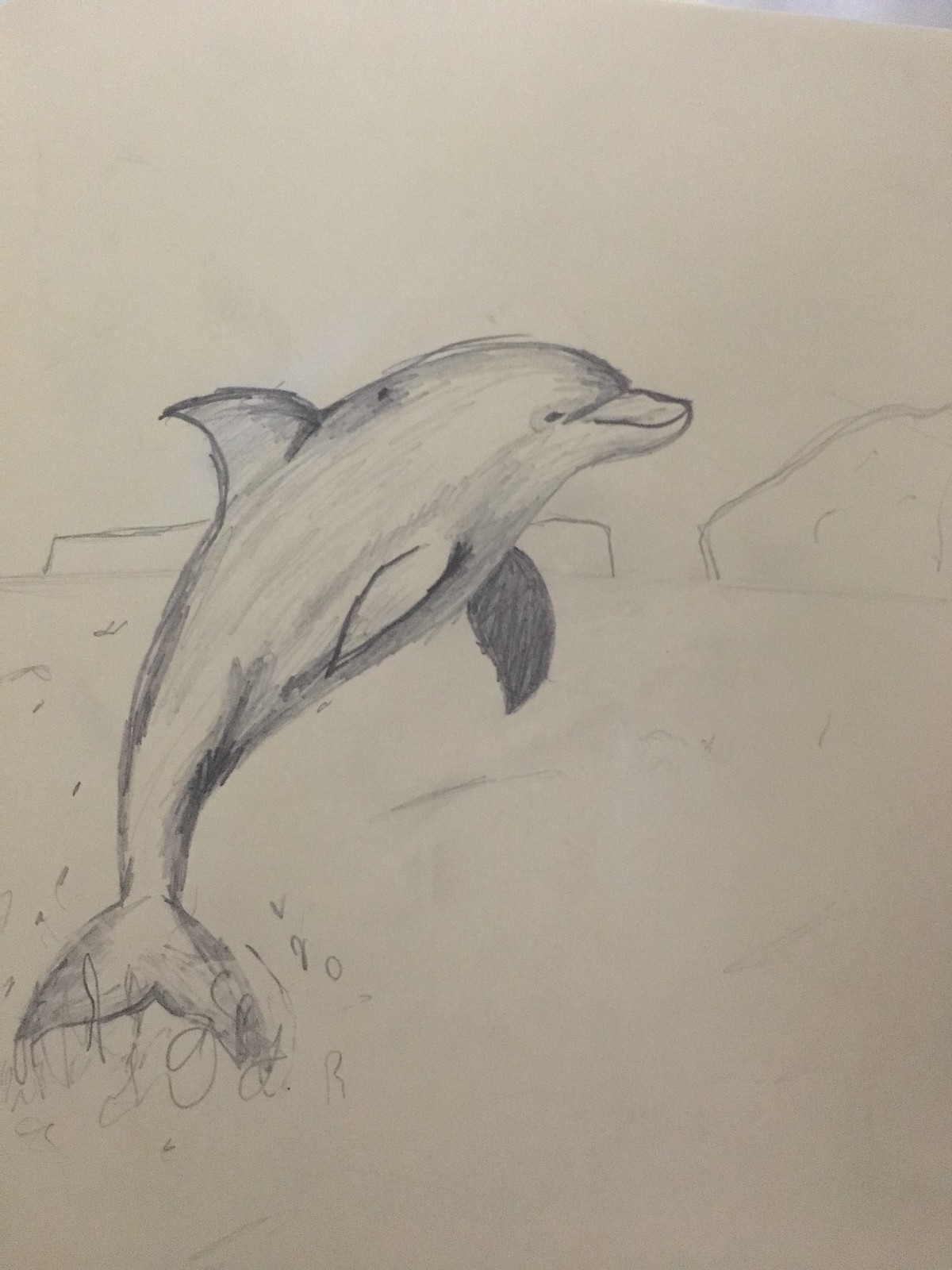A lightly detailed pencil sketch on tan paper captures a dolphin playfully emerging from the water. The dolphin, depicted with a gentle smile, displays intricate shading on its fins and snout, bringing a touch of realism to its form. In the background, faint outlines hint at surrounding rocks, while bubbles in the lower left corner indicate the dolphin's dynamic leap. Despite its simplicity, the artist adeptly portrays the natural shadows and contours of the animal, making the dolphin appear lifelike even with minimal backdrop details.